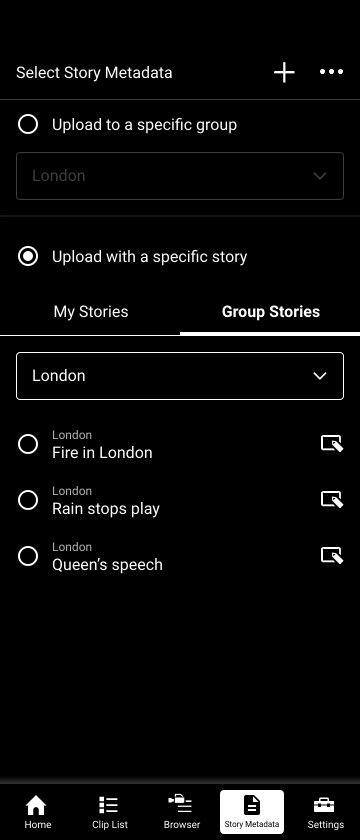The image displays a user interface with a predominantly black background. At the top left, there is a title labeled "Select Story Metadata." To the right of this title, a plus symbol is present, followed by a horizontal ellipsis. Below this section, a black circle with a white border contains the text "Upload to a specific group." Beneath this, there is a drop-down menu with gray borders labeled "London."

Further down, there is another circle similar to the first, but filled in, which is labeled "Upload with a specific story." Below this, the interface presents two sections: "My Stories" on the left and "Group Stories" on the right. A thin white line is placed under "My Stories" and a thick white line under "Group Stories."

Under these sections, there is another drop-down menu labeled "London." Below this, a black circle with a white border states "London fire." Immediately following are more circles with corresponding labels: "London rain stops play," and "London Queen's Speech." The remaining bottom portion of the image is an empty black area.